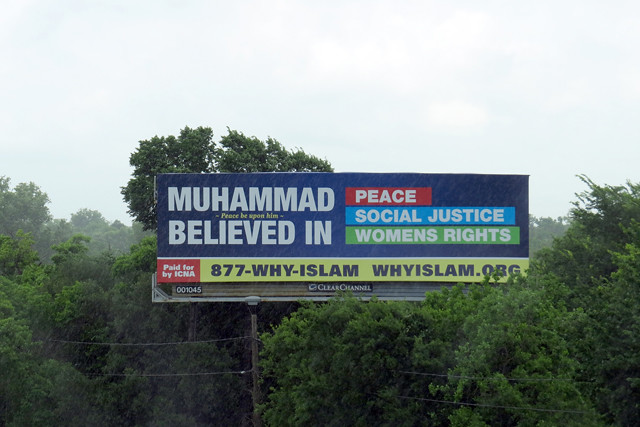The photograph features a billboard elevated among verdant, green trees. The billboard is notably high, as evidenced by the power lines running below it. The sky above is cloudy, with a substantial amount of sky visible above the tree line.

The billboard itself presents a powerful message, boldly stating, "Muhammad believed in peace, social justice, women's rights." This message is sponsored by ICNA, indicated in the lower left corner. Below the endorsement, a contact number, 877-Y-ISLAM, and a website, Yislam.org, are provided for further information.

The design of the billboard is visually striking, with the upper portion featuring a blue background, while the lower portion transitions into red and yellow hues, enhancing the overall impact of the message.